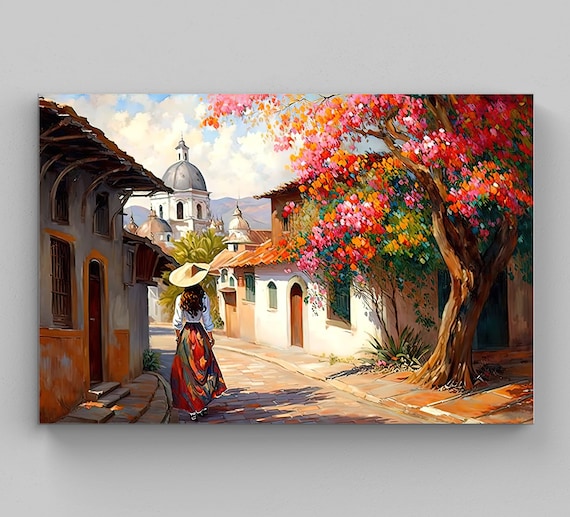The image depicts a vibrant, watercolor painting mounted on a slightly gray wall. Dominating the scene is a woman seen from behind, walking down a narrow, brick street reminiscent of old European or Spanish-style architecture. She wears a white long-sleeved blouse, an ankle-length multicolored skirt, and a tan hat atop her long brunette hair. As she proceeds toward a domed, chapel-like building in the distance, adobe-like buildings with orange roofs and steps flank her path. To her right, a mature tree with a riot of pink, red, orange, and green foliage provides a burst of color against the background of a cloudy sky. Sporadic weeds grow near the base of the building to her right, adding a touch of authenticity to the picturesque and serene setting.